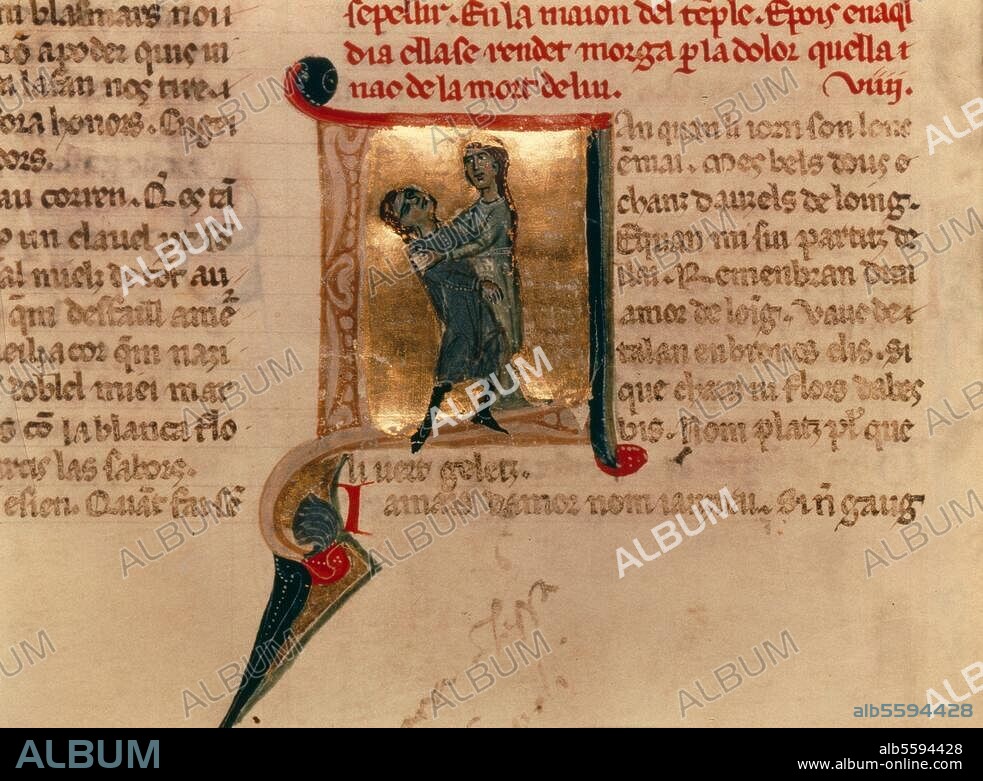The image showcases an ancient-looking artwork centered on what appears to be old parchment paper, with intricate and ornate gold, red, and green illustrations. The central artwork depicts a woman, seemingly adorned with a crown, embracing a man with dark eyes who appears to be falling back. This scene is framed by gold foil and elaborate decorative strokes in red and teal. The parchment background features gold-brown text columns on both sides and additional red script above the artwork, giving the impression of medieval manuscript styling, possibly created by monks around the 1100s or 1200s.

Across the image, the word "album" is repeatedly watermarked in varying degrees of opacity, with some instances being transparent and others white. At the page's bottom, a dark blue bar features the word "album" on the left and text reading "alb5594428 www.album-online.com" on the right. The overall impression is of a historical text infused with an artistic illustration and contemporary digital watermarks.